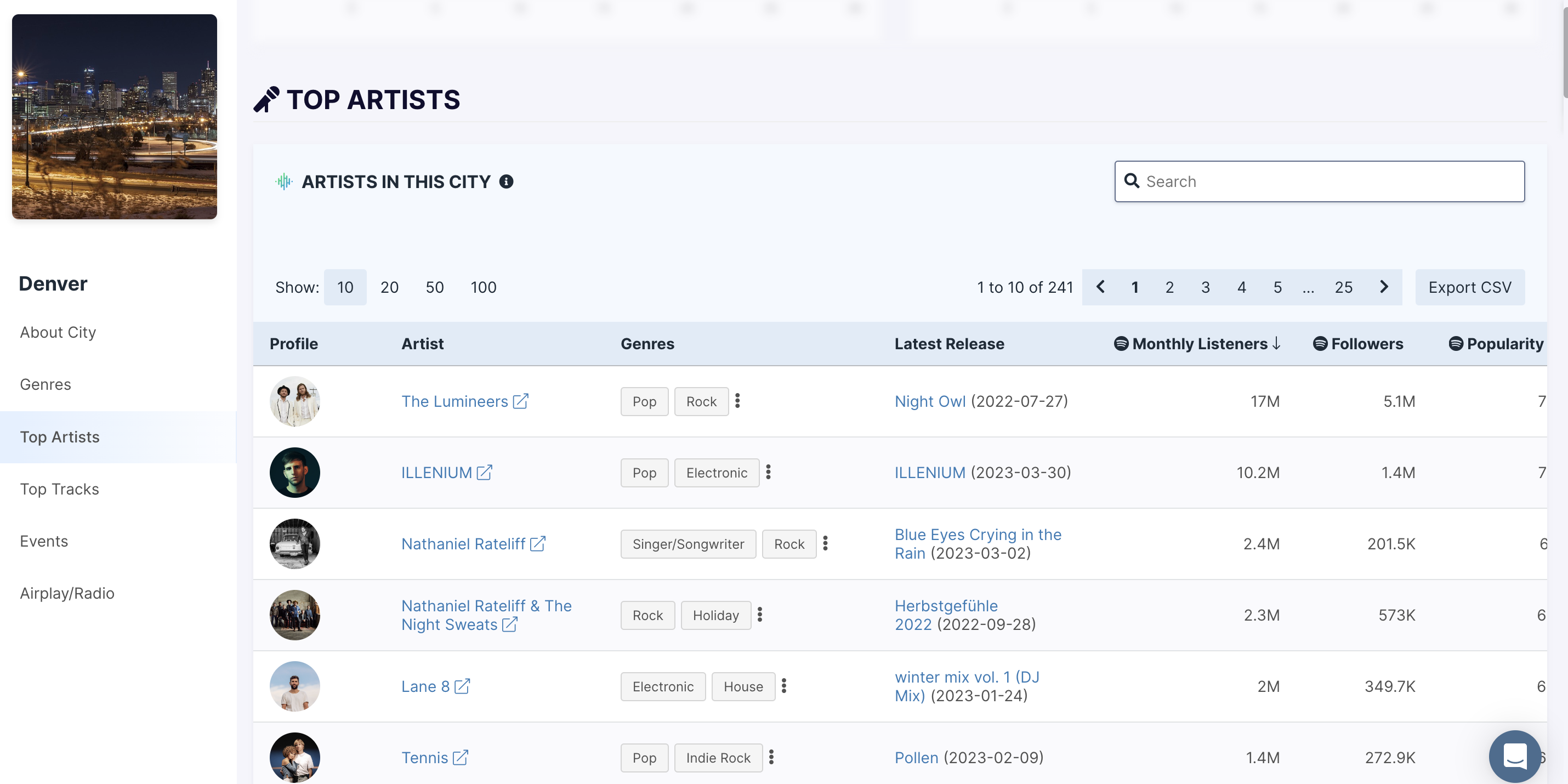The image showcases a detailed list of artists associated with a specific area. On the far right of the screen, there is a square picture of a cityscape at night, foregrounded by a yellowish-hued park, with skyscrapers towering in the background. Directly below this image, it reads "Denver" and includes various categories such as "City," "Genres," "Top Artists," "Top Tracks," "Events," and "Airplay/Radio." These categories are listed in a white vertical bar on the left side.

To the right of this menu, the screen's background is a light bluish-gray. At the top right section, the header "Top Artists" is displayed in black text, accompanied by a small microphone icon.

Below this header, the image highlights the top 10 artists from this city, complete with their profile pictures, monthly listeners on Spotify, followers, popularity rating, and genre. 

- **The Lumineers**: Genre - Pop rock. Latest release - "Night Owl". Monthly listeners - 17 million. Followers - 5.1 million. Popularity - 7.
- **Illenium**: Genre - Pop electronic. Latest release - "Illenium". Monthly listeners - 10.12 million. Followers - 1.4 million. Popularity - 7.
- **Nathaniel Rateliff**: Genre - Singer-songwriter/Rock. Latest release - "Blue Eyes Crying in the Rain". Monthly listeners - 2.4 million. Followers - 201,000. Popularity - 6.
- **Nathaniel Rateliff & The Night Sweats**: Genre - Rock. Latest release - "Holiday" (in German). Monthly listeners - 2.3 million. Followers - 573,000. Popularity - 6.
- **Lane 8**: Genre - Electronic/House. Latest release - "Winter Mix Volume 1". Monthly listeners - 2 million. Followers - 349.7 thousand. Popularity - 6.
- **Tennis**: Genre - Pop Indie Rock. Latest release - "Pollen". Monthly listeners - 1.4 million. Followers - 272.9 thousand. Popularity - Not fully visible due to an icon overlap.

The overall presentation is organized and contains essential metrics for each artist, providing a comprehensive overview of the music scene in Denver.